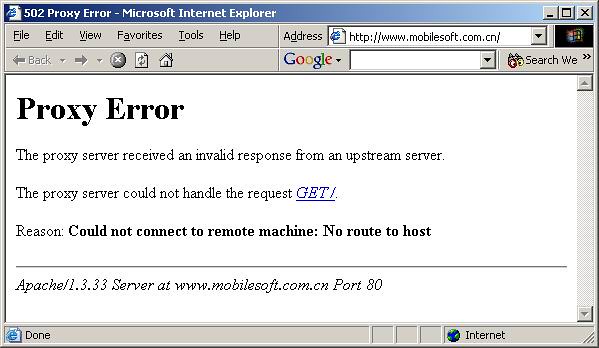The image depicts an old-fashioned Windows screen displaying an error message in Microsoft Internet Explorer. At the top, it reads "502 Proxy Error - Microsoft Internet Explorer," and features the classic blue 'E' icon with a blank page beside it. The browser includes standard menu options: File, Edit, View, Favorites, Tools, and Help. To the right, there's an Address bar containing the URL "http://www.mobilesoft.com.cn/". Below that, typical browser navigation buttons are present, including Back, Forward, Cancel, Refresh, and Home.

In the main part of the window, the error message "Proxy Error" is prominently displayed in bold. The detailed error message reads: "The proxy server received an invalid response from an upstream server. The proxy server cannot handle the request GET." It continues, "Reason: Cannot connect to remote machine: No route to host," with "cannot host" emphasized in bold. A dividing line follows, noting "Apache 1.3.33 Server at www.mobilesoft.com.cn Port 80".

Additionally, there is a Google search bar, and at the bottom of the screen, the status displays "Done" in the bottom left and a globe icon with "Internet" in the bottom right.